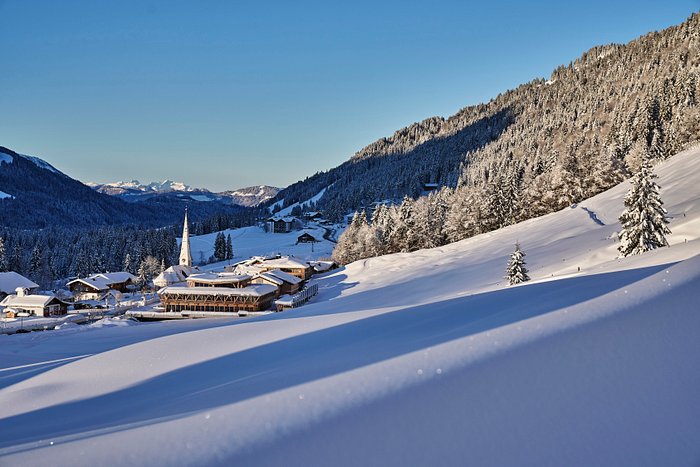This image captures a picturesque, snow-covered village nestled in the mountains on a sunny, cloudless day. On the right side of the photograph, a large hill or mountain ascends from left to right, its front half blanketed with fresh snow while the back is densely forested with evergreen trees. At the base of this hill, the quaint village features a collection of brown houses, their roofs heaped with snow. Dominating the village skyline, a white church with a tall steeple stands prominently in the center. To the left, the scene extends to distant, snow-capped mountains. The sky above is a clear, vibrant blue, intensifying the serene and pristine beauty of this secluded village.